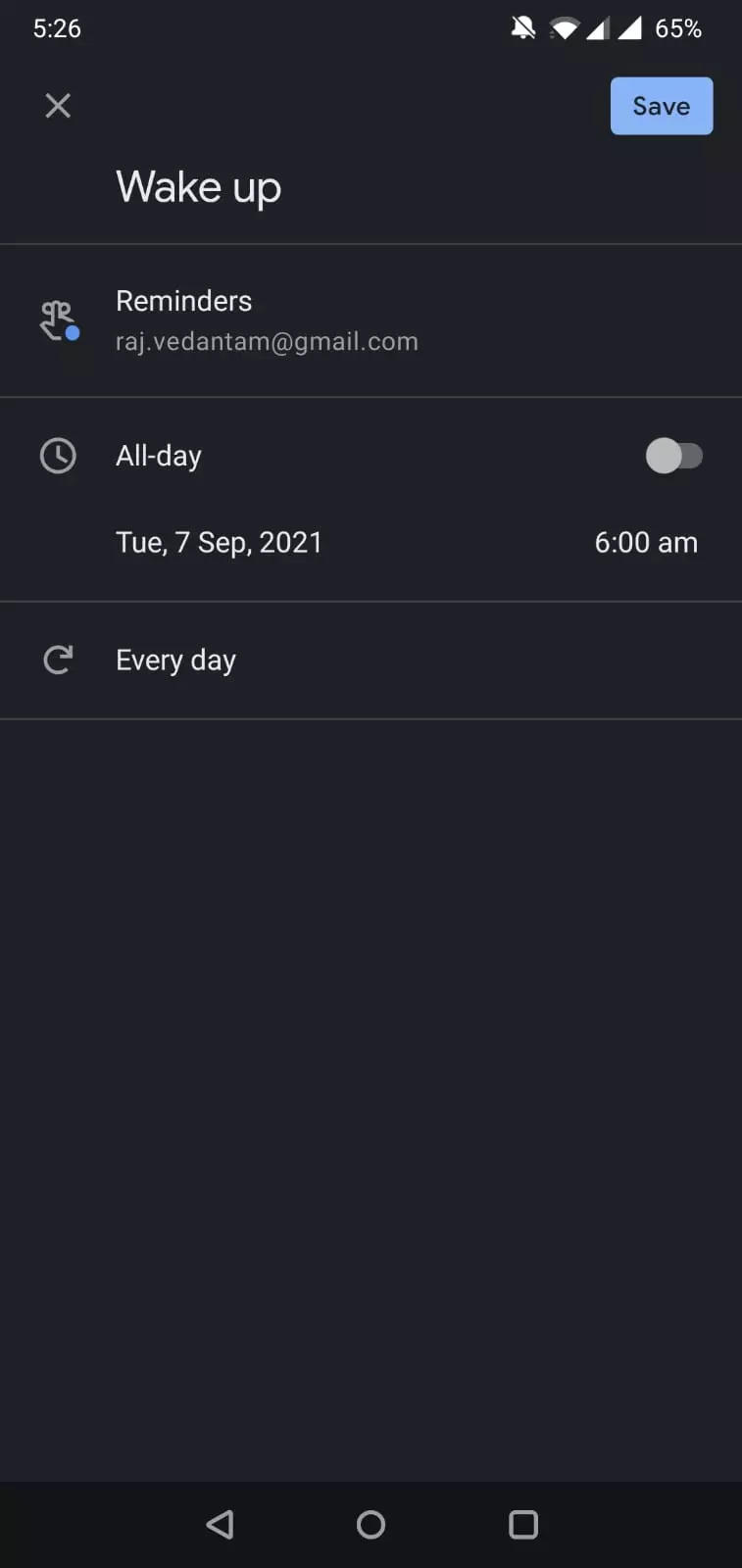Screenshot of a smartphone screen captured in vertical orientation. 

- **Top Section:**
  - **Left Side:** In the upper left corner, the time is displayed in white: "5:26".
  - **Right Side:** Icons displayed in white include a muted bell, a Wi-Fi signal, various triangle symbols, and a battery icon with 65% remaining.

- **Middle Section:**
  - Below the time, a gray 'X' symbol is visible, followed by the text "Wake Up" in white.
  - A line separates this from the following section.

- **Reminders Section:**
  - The header "Reminders" is displayed, accompanied by a small icon featuring a blue circle.
  - Below it, the email "raj.vedantam@gmail.com" is listed.
  - Another line separates the above from a section featuring a clock symbol and the text "All Day", followed by "Tuesday, 7 September, 2021, 6 a.m.", indicating an active reminder that can be toggled on or off (currently off).

- **Additional Options:**
  - Following another line, a reverse arrow icon is shown alongside the text "Say every day".

- **Bottom Section:**
  - At the very bottom of the screen, three navigation icons are displayed: a triangle, a circle, and a square.

The detailed visual elements indicate a typical reminder notification interface with options for managing the reminder frequency and activation.